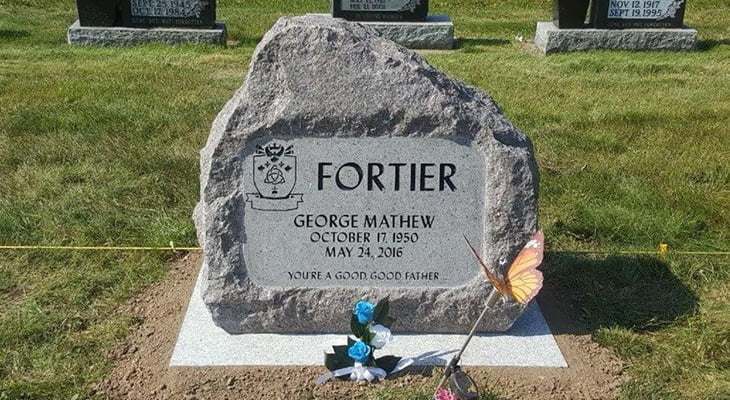This outdoor photograph depicts a gravesite with a grey, irregularly shaped tombstone crafted from granite. The text inscribed on the tombstone reads: "Fortier, George Matthew, October 17, 1950, May 24, 2016. You are a good, good father." It sits atop a white marble base surrounded by brown soil. In front of the tombstone, there are flowers—a white one and two small blue ones, centrally placed with a ribbon tied around them. Additionally, there is a stick with a butterfly figure pierced into the ground to the right. The background displays a grassy area with the bottom parts of three other faintly visible tombstones, bathed in sunlight. There's also an unmarked crest symbol on the tombstone, possibly a triple-point or Möbius line, and behind the gravesite, a yellow caution line can be seen, indicating potential recent burial activity.